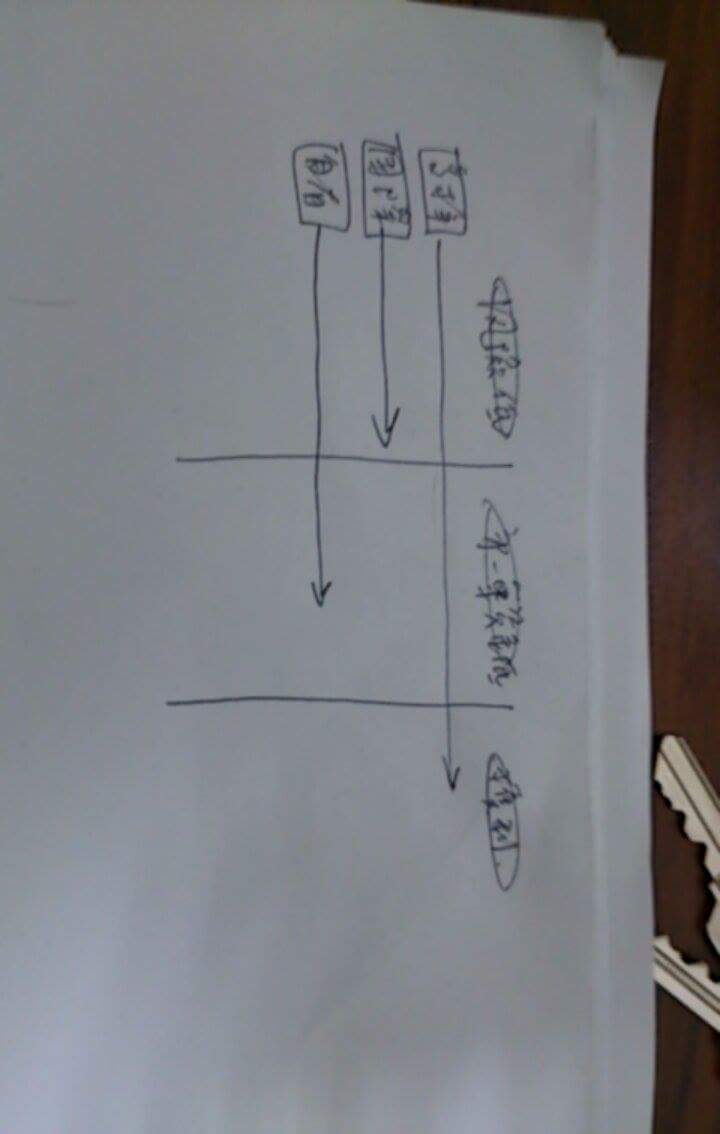A slightly angled photograph captures a piece of white paper placed on a dark reddish-brown table. The paper, positioned in a vertical rectangle orientation with the top facing sideways, showcases handwritten sketches and markings that require a head tilt to read correctly. Among the visible items in the scene are the edges of two house keys lying partially atop the paper.

The main focus of the photograph is the series of sketches: three small hand-drawn rectangles aligned vertically on the left side of the paper, each with an arrow extending to the right at varying lengths. These arrows intersect two horizontal lines stretching across the paper. Additionally, three oval shapes are situated on the right side, containing markings that resemble intricate or Asian-like characters. The detailed and somewhat cryptic nature of the sketches suggests a complex or conceptual diagram that invites closer inspection.